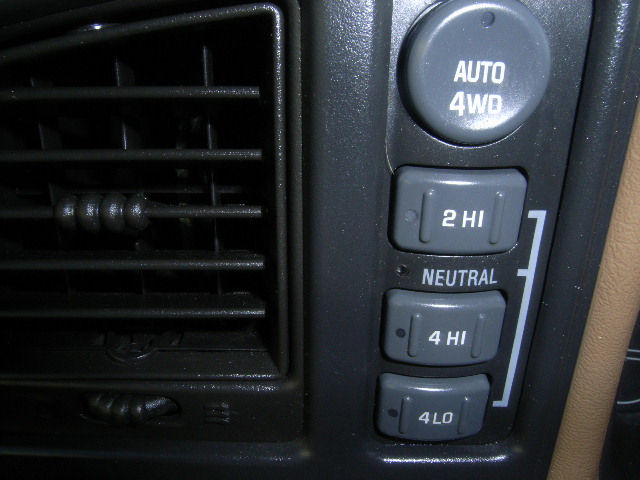This close-up image captures the detailed interior of a vehicle, focusing on an air conditioning vent and an adjacent control panel. The vent is black and has a shiny, plastic appearance. To its right, the control panel features four buttons with a distinct arrangement and labeling in white letters. At the top is a circular gray button labeled "Auto 4WD." Below it, there are three rectangular gray buttons: the first labeled "2HI," the middle space indicating "Neutral," the third labeled "4HI," and the fourth button labeled "4LO." A light tan trim runs parallel to the black surface of the vent, providing a subtle contrast to the dark tones of the vent and panel.